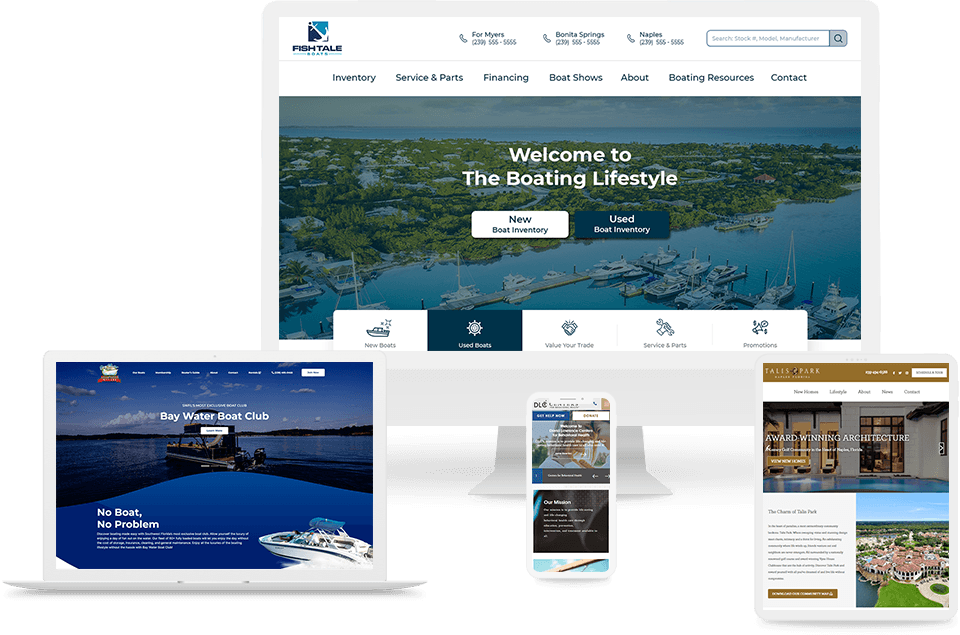The image depicts a variety of electronic devices showcasing different websites. Dominating the background, positioned top center, is a white desktop computer monitor. The screen displays a webpage titled "Fishtail," distinguished by an anchor logo on the top-left corner. Prominently featured in the middle of the screen is the welcome message, "Welcome to the Boating Lifestyle," followed by buttons labeled "New Boat Inventory" and "Used Boat Inventory," with the latter being highlighted in blue. At the bottom of the screen, there are images accompanied by labels such as "New Boats," "Used Boats," "Value Your Trade," "Service and Parts," and "Promotions."

In the foreground, on the left side, sits a white laptop. Its screen shows a website for "Baywater Boat Club," featuring the slogan "No Boat, No Problem," with some unreadable smaller text at the bottom. The background image on this site showcases a boat with another boat visible at the bottom right.

Centrally located in the foreground is a white smartphone, though the text on its screen is too minute to discern. On the right-hand side is a white tablet, displaying a webpage with the headline "Award-Winning Architecture." Behind this text is an image depicting a house or apartment, complete with a pool. Beneath this banner, there is more illegible text, and to the right, an image that suggests a college.